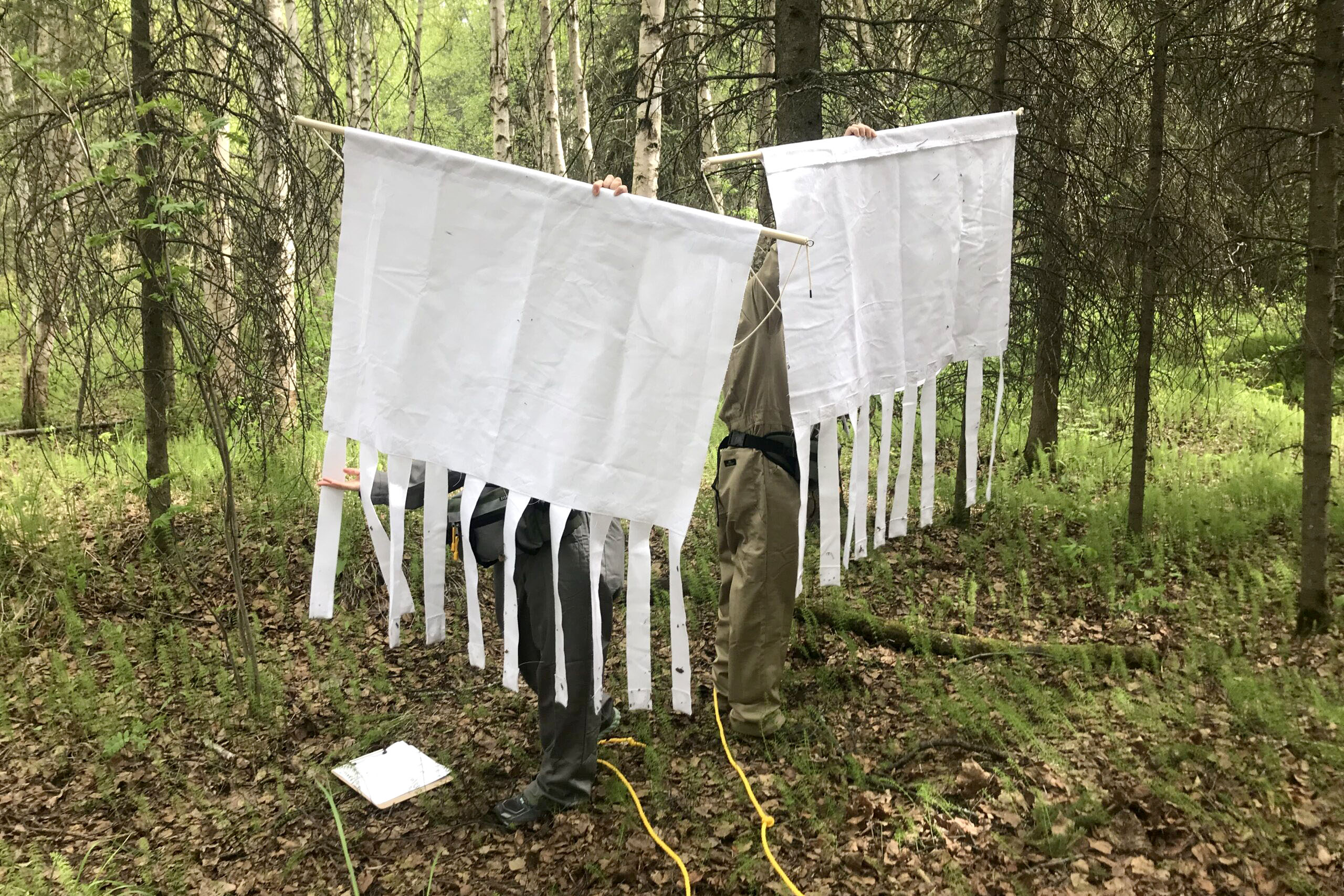In this vibrant forest scene, tall and slender white birch trees dominate the left side, with smaller black-trunked trees scattered on the right. The forest floor is a rich mix of brown leaves interspersed with sprouting green weeds. Two yellow ropes lie across the center ground. Amid this natural setting, two individuals stand side-by-side, each holding up a large, solid white banner mounted on thin tan-colored poles, their faces obscured by the cloth. The banners feature frilly strips hanging from the bottom, reminiscent of medieval designs. The person on the left is dressed in dark grey, while the person on the right wears khaki. Nearby, on the forest floor to the left, a white notepad is visible.